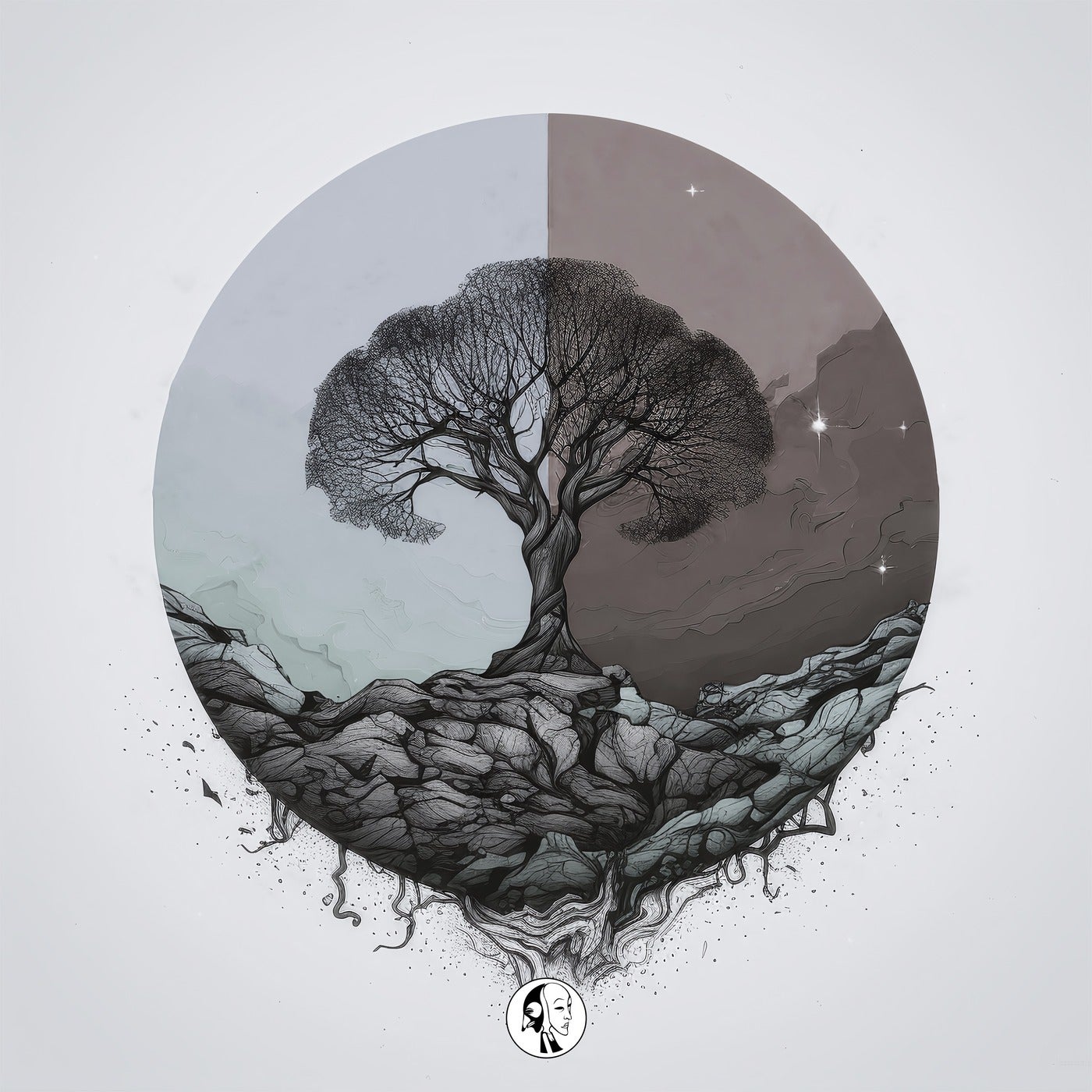The image features a central circle set against a gray background, with the circle divided into a lighter left half and a much darker right half, potentially symbolizing day and night. Placed in the middle of this circle is an intricately detailed etching of an old tree, appearing almost ginkgo leaf-like in its wispy, willowy branches. The tree is rooted atop a mound comprised of numerous small rocks, scattered in a valley-like formation. Notably, the tree's entangled roots burst out from the bottom of the circle, protruding into the surrounding space.

The darker right side of the circle displays a night scene, complete with scattered white twinkling stars and dark clouds. In contrast, the left side, though also cloudy at the bottom, remains lighter, suggesting it is not nighttime yet. Below the circular etching, there is a small white circle containing a logo: a bifurcated face. On the left, the face resembles a penguin or a bird with a beak, while on the right, a more human face frowns. This monochromatic artwork, rich with texture and contrasts, not only emphasizes the tree growing resiliently among rocks but also hints at depth through the inclusion of changing skies and an abstract emblem.